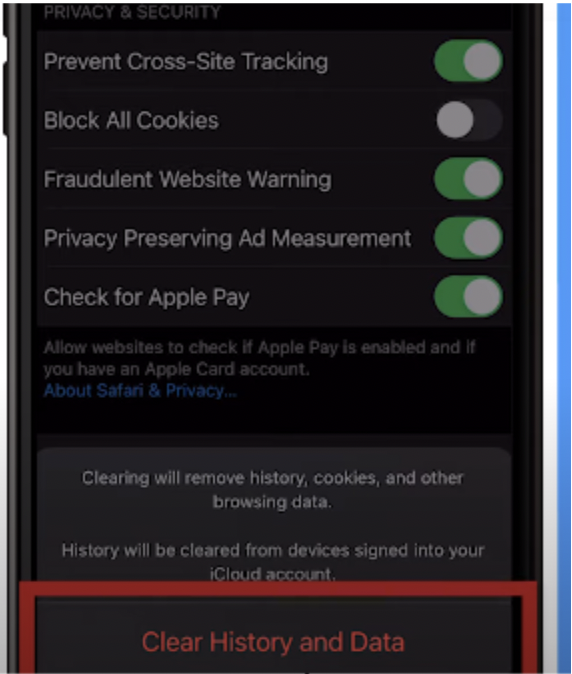This image features a detailed view of a privacy and security settings screen. At the top, the heading "Privacy & Security" is prominently displayed. Below it, five options are sequentially listed, each with a toggle button on the right. Among these options, four are toggled on, indicated by a green and white switch. The options are as follows:

1. Block All Cookies (toggled on)
2. Prevent Cross-Site Tracking (toggled off)
3. Fraudulent Website Warning (toggled on)
4. Privacy-Preserving Ad Measurement (toggled on)
5. Check for Apple Pay (toggled on)

Underneath the last option, a gray text snippet reads, "Allow websites to check if Apple Pay is enabled and if you have an Apple Card account."

Below this, in blue text, there is a link titled, "About Safari & Privacy."

Further down, a section notes, "Clearing will remove history, cookies, and other browsing data. History will be cleared from devices signed into your iCloud account."

At the very bottom of the screen, there is a red button outlined with a red border that says, "Clear History and Data."

On the right side of the image, there’s a background that transitions from light gray at the bottom (covering about 10%) to white at the top, forming a narrow, vertical, rectangular shape. Adjacent to this, a consistent blue background extends from top to bottom, completing the visual layout.